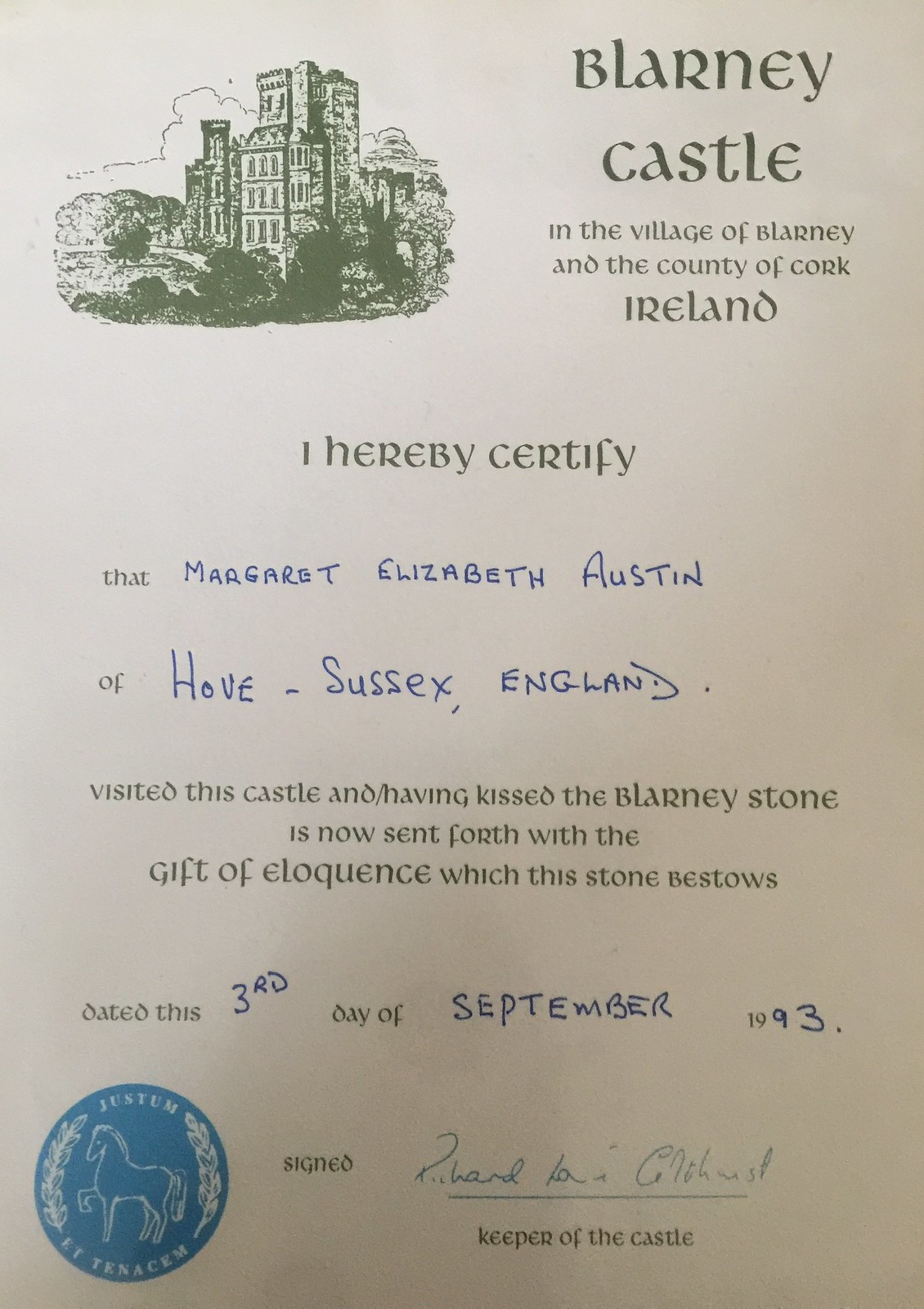This is an image of a Certificate of Authenticity from Blarney Castle in the village of Blarney, County Cork, Ireland. The document, set against a cream-colored background with primarily dark green text, features an old-school drawing of the castle and its surrounding landscape in the upper left corner. Adjacent to this illustration, it reads "Blarney Castle in the village of Blarney in the county of Cork, Ireland." Centered beneath this, in dark green text, it certifies that "Margaret Elizabeth Austin of Hove, Sussex, England visited this castle and, having kissed the Blarney stone, is now sent forth with the gift of eloquence which the stone bestows."

The certificate is dated the "3rd day of September 1993," with the date handwritten in blue ink. In the bottom left corner, there is a small blue circular seal featuring the white outline of a horse, accompanied by the Latin phrase "Justum et Tenacem." The document concludes with the signature of Richard (illegible last name), identified as the Keeper of the Castle. The certificate is a cherished memento for visitors to affirm their visit and the unique experience at Blarney Castle.